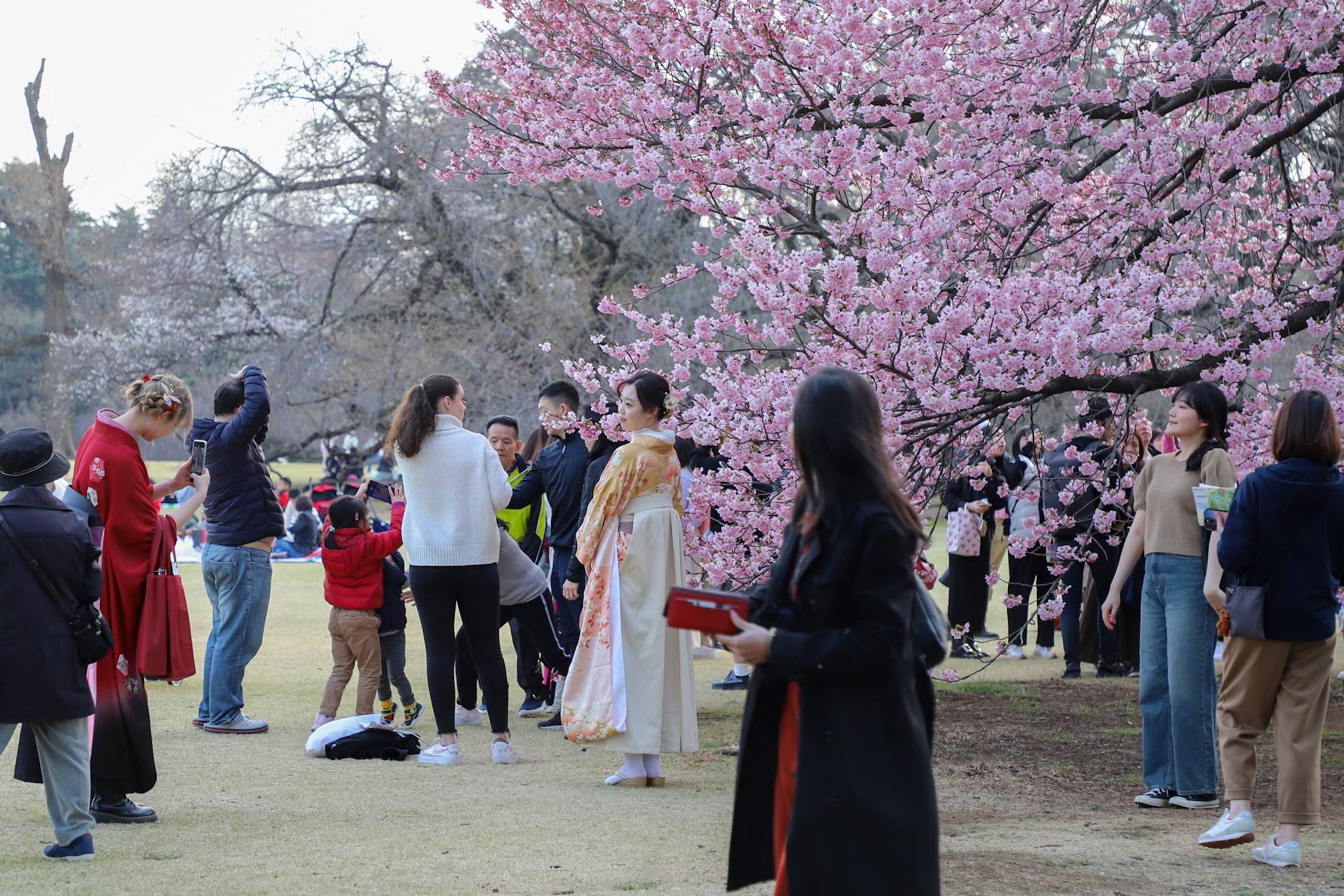The image depicts an outdoor gathering likely during a cherry blossom festival in a park in Japan. Central to the scene is a large tree adorned with vibrant pink cherry blossoms, attracting numerous individuals who are posing for photographs. Among them is a Japanese woman dressed in a traditional kimono, which features an off-white back and an orange floral pattern on the front. She accessorizes with white socks, traditional sandals, and has her hair pulled back with a floral hairpin. The overall atmosphere suggests a chilly day as many attendees are wearing coats. People of all ages, including children and adults, are present, with some using cell phones to capture the scenic beauty and others simply observing. In the background, additional trees stand, yet to bloom, framing the main focus—the striking cherry blossom tree.